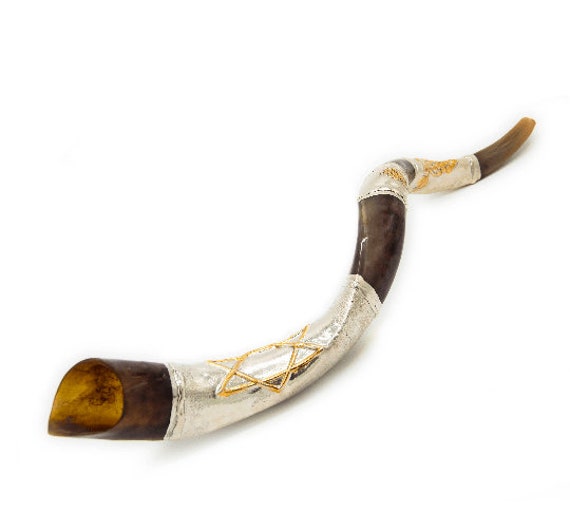The image depicts an ancient, snake-like musical instrument, resembling a horn or trumpet. The object is a blend of earthy browns and silver, making it appear somewhat transparent in spots. The instrument is segmented with alternating brown and silver sections, giving it a layered look. The silver segments are reflective, almost foil-like, and feature intricate designs. Notably, there is a prominent Star of David on the foremost silver segment. The horn curves sinuously with two distinct bends and culminates in a pointed, brown mouthpiece. The background of the image is stark white, offering no context for scale but highlighting the object's detailed craftsmanship and antique appearance.